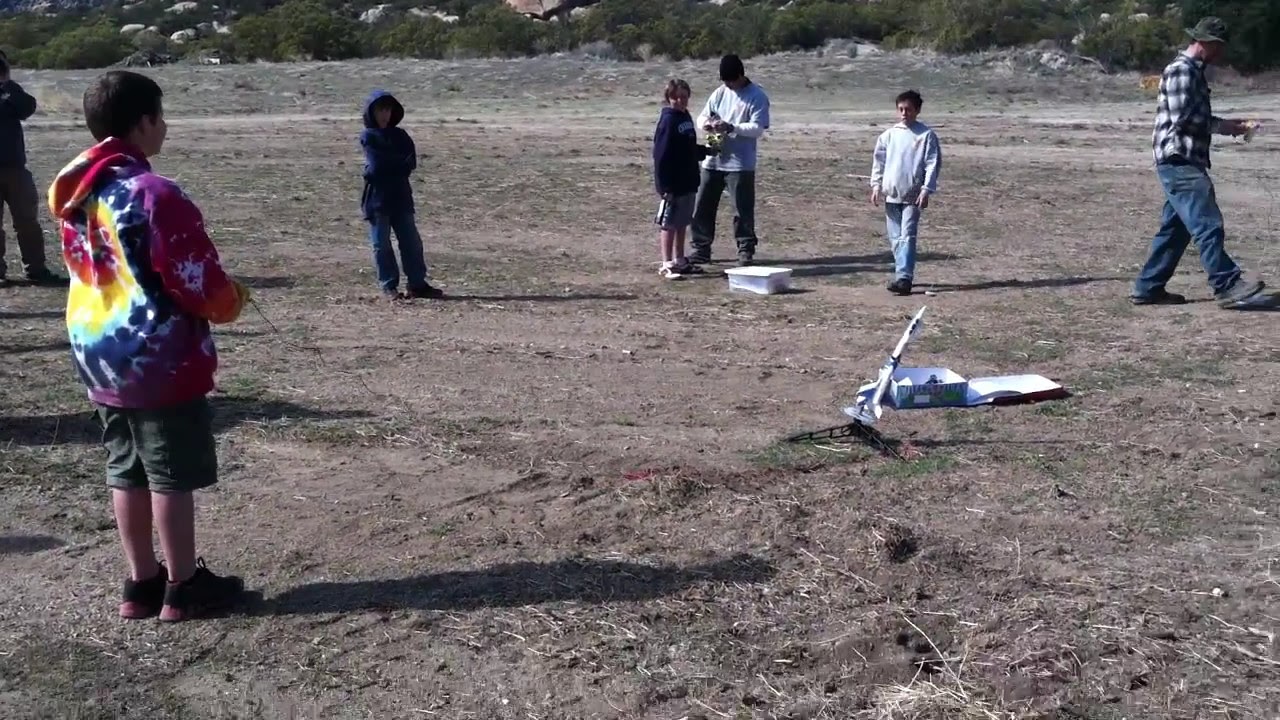In this vivid outdoor scene, a group of young boys and one adult male are gathered in a dry, barren landscape, reminiscent of a desert. The adult male, who's outfitted in a black and white plaid shirt, jeans, grey shoes, and a stylish black Panama hat, is assisting the children as they prepare to launch a firework. The firework stick is firmly planted in the ground, acting as the focal point around which the activity revolves. Scattered boxes lie nearby, likely containing more fireworks or related equipment.

The boys, aged roughly between 10 and 12, are dressed in various brightly colored garments, creating a striking contrast against the tan and brown earth. One boy stands out with his multi-colored tie-dye hoodie, paired with shorts and sneakers, and he holds a controller, possibly for the firework. Other boys are clad in hoodies of different shades—white, grey, black—along with jeans or shorts. They all seem to be moving around the central figure of the firework, some appearing busy with preparations, while others stand back, watching with crossed arms.

In the distance, some sparse trees and a couple of rustic buildings are visible under the bright daytime sky, adding a sense of depth to the otherwise flat field. The scene captures a moment filled with anticipation and teamwork amidst a stark, open setting with no text or signs in view, emphasizing the raw, unembellished nature of the location.